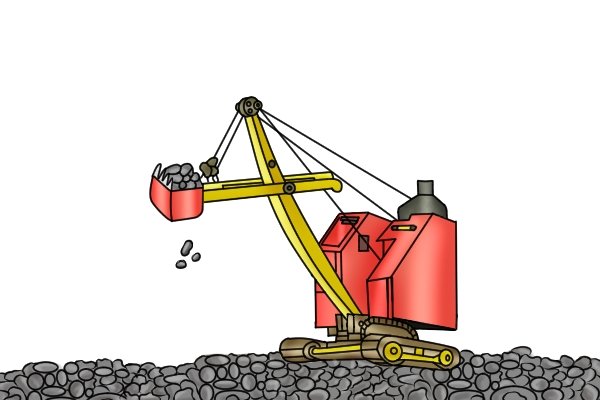The image features an amateurish, hand-drawn or digitally-created cartoon of a construction site set against a stark white background. At the heart of the scene is an old-fashioned crane with a wire-driven mechanism, positioned centrally. This crane is red in color, with brown tracks and wheels, and has multiple yellow handles or arms extending upwards. The crane is actively scooping up gray and occasional green stones from a ground covered entirely in rock and gravel, which are depicted in various shades of gray. The red bucket of the crane, adorned with white teeth, is in the upper left corner, lifting rocks. The base on which the crane rests is a dark gold or brownish hue, contrasting with the abundance of stones scattered around. The illustration conveys an art style akin to a basic and unsophisticated drawing, emphasizing the simplicity and roughness of the composition. Despite the crude execution, the detailed elements and specific colors draw the viewer into the construction site setting, where the machinery tirelessly gathers the scattered stones.